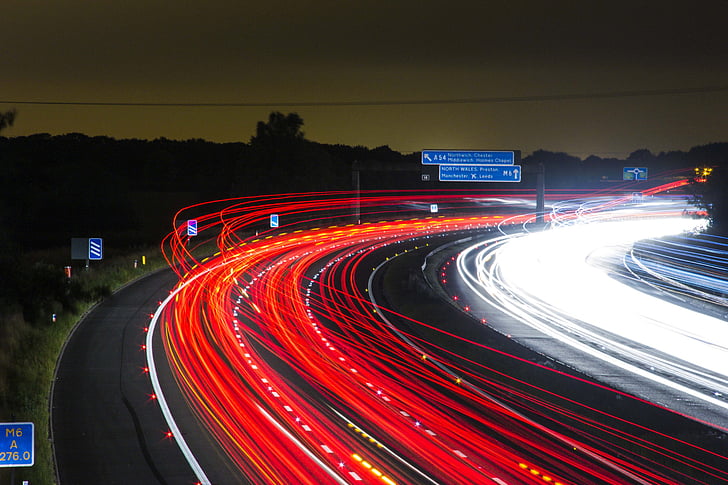This image depicts a night-time highway captured with time-lapse photography. The scene is bathed in streaks of light, emphasizing the speed and movement of traffic. On the left side of the highway, a series of red streaks represents the taillights of vehicles traveling away, while the right side is dominated by white streaks from oncoming headlights. The red and white light trails curve in a semicircular pattern, resembling an 'S' shape, which overlays the black roadway marked with white lane lines.

In the background, dark silhouettes of trees and a light gray overpass adorned with multiple signboards set the scene. The sky above transitions from dark gray to black, adding to the night-time ambiance. The grassy verge on the left side of the highway is dotted with more road signs indicating directions and exits. The image suggests a busy roadway, possibly in a European country, inferred by the unfamiliar numerical signs and directional indicators. The high-speed appearence of the vehicles is achieved through long exposure photography, capturing the essence of motion and the bustling activity of the highway at night.